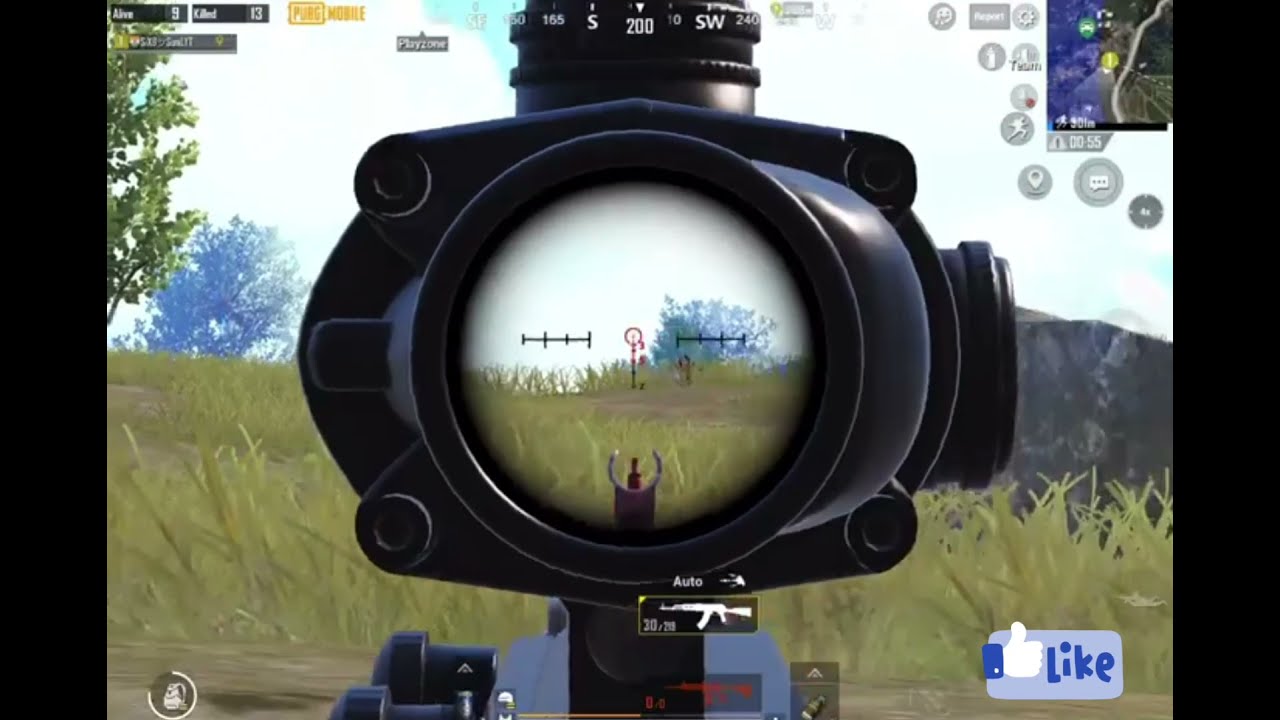The image is a detailed screenshot from a sniper shooting video game, captured from the player's point of view. The main focus is a sniper scope centered on the screen, with a small red reticle inside a black circular frame. The scope features horizontal and vertical lines for precision aiming. In the distance, the view includes a green tree against a gray sky, and green grass below. At the top center, there's a compass showing directional headings from south to southwest, with a degree reading of 200. The upper-right corner displays a map indicating the player's location and various game functions. In the bottom-right corner, there's a blue rectangle with a thumbs-up icon labeled "like," suggesting the game is being live-streamed or recorded for viewers. The image is bordered by thin vertical black rectangles on each side, framing the in-game screenshot.